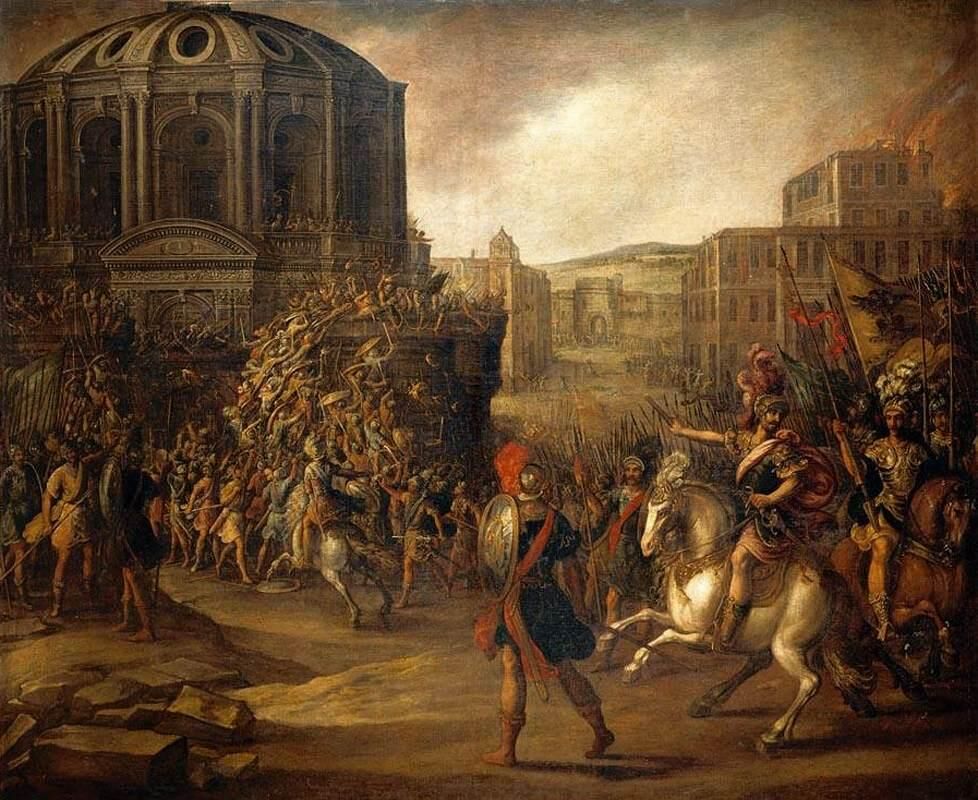In this large square Renaissance-style painting, a vivid and chaotic battle scene unfolds, dominated by warm brown hues that give the image a somber tone. In the upper left corner stands a prominent two-story domed building, characterized by its arched windows and stone architecture. Surrounding this structure is a teeming mass of people, seemingly clambering over each other in a frantic surge.

In the foreground, the central figure is a soldier adorned in a black gown, brandishing a large gold shield and distinguished by red feathers on his helmet and a red scarf. He appears to be leading a procession of similarly outfitted soldiers. Prominently featured beside him is a golden horse rearing on its hind legs, adding to the scene's dynamic intensity. Both soldiers and fighters, equipped with shields and spears, march behind this pair, underscoring the painting’s martial theme.

On the right side of the image, another man on a white horse points toward the tumultuous crowd amassed around the grand building. Behind him, a contingent of soldiers on horseback brandish flags, indicating the organized martial force involved in the conflict. This detailed depiction, replete with soldiers in helmets decked with feathers and wielding various weapons, along with the presence of multiple stone buildings in the background, evokes the grandeur and chaos of a historic battle, potentially alluding to confrontations from the Roman Empire or a similar epoch.